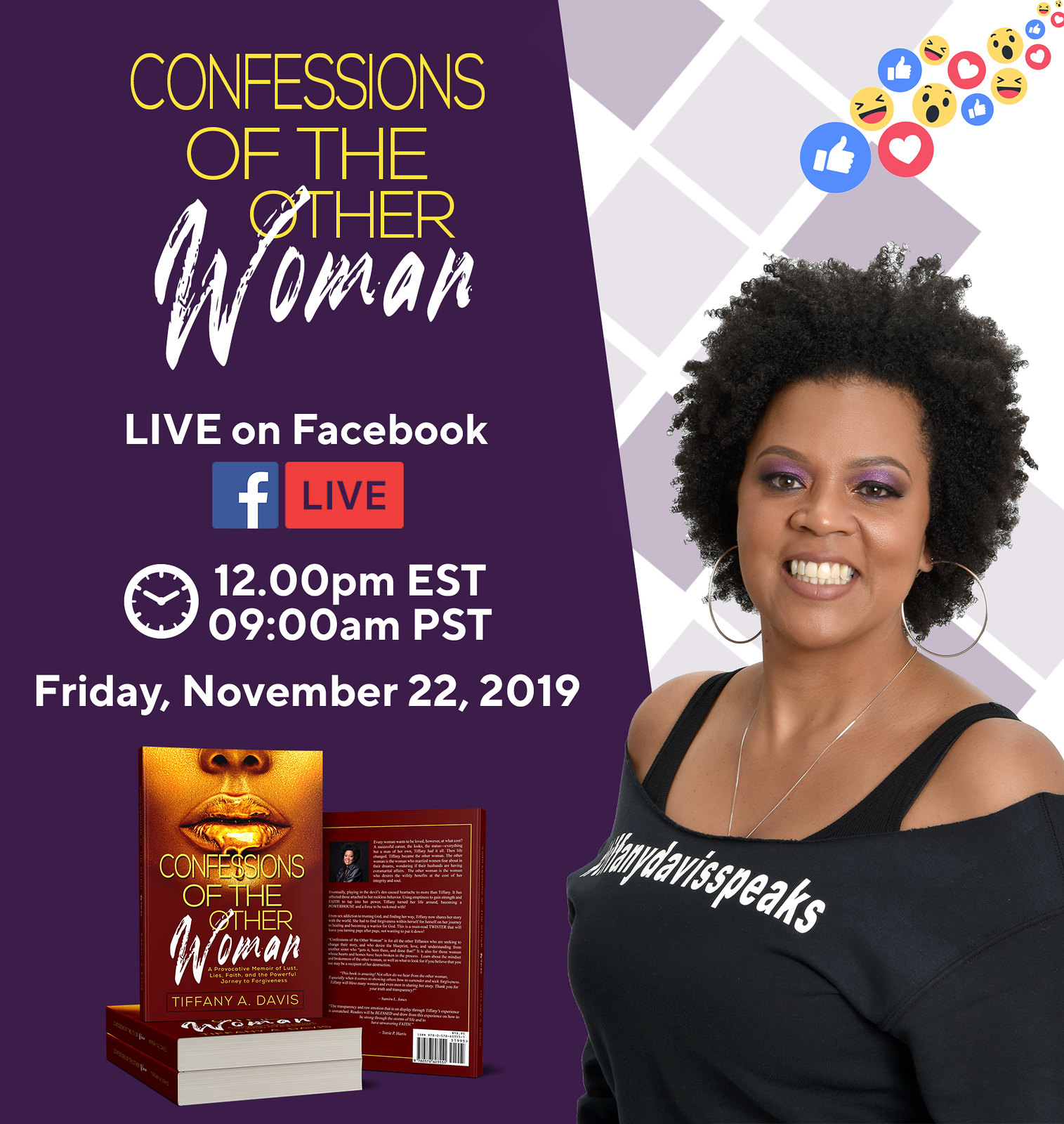This advertisement for the book "Confessions of the Other Woman" prominently features a vibrant and engaging layout. On the left-hand side, a purple background with bold yellow and white text announces the book's title, "Confessions of the Other Woman." Below this, it details an event "Live on Facebook" with the Facebook logo and a red box indicating "Live" in blue letters. An image of a clock signifies the schedule for the event: 12 p.m. Eastern Time and 9 a.m. Pacific Time on Friday, November 22, 2019. Accompanying this information is a visual of two stacked books showcasing both the front and back covers. The front cover displays a close-up of a woman's gold lips, while the back reinforces the book's title in text. Surrounding the event details are engaging emojis such as smiley faces, shocked expressions, hearts, and thumbs-up icons.

To the right, a woman, presumably the author, captures the viewer's attention. She has short, curly black hair styled into an afro and wears purple eyeshadow. Her wide smile reveals big, white teeth, and she is adorned in a black off-the-shoulder shirt layered over a black tank top, with large hoop earrings and a silver necklace. The shirt features the text "Manny Davis Speaks" in white lettering. Her pleasant demeanor and confident image enhance the advertisement's appeal, inviting viewers to engage with the live event and explore her book.